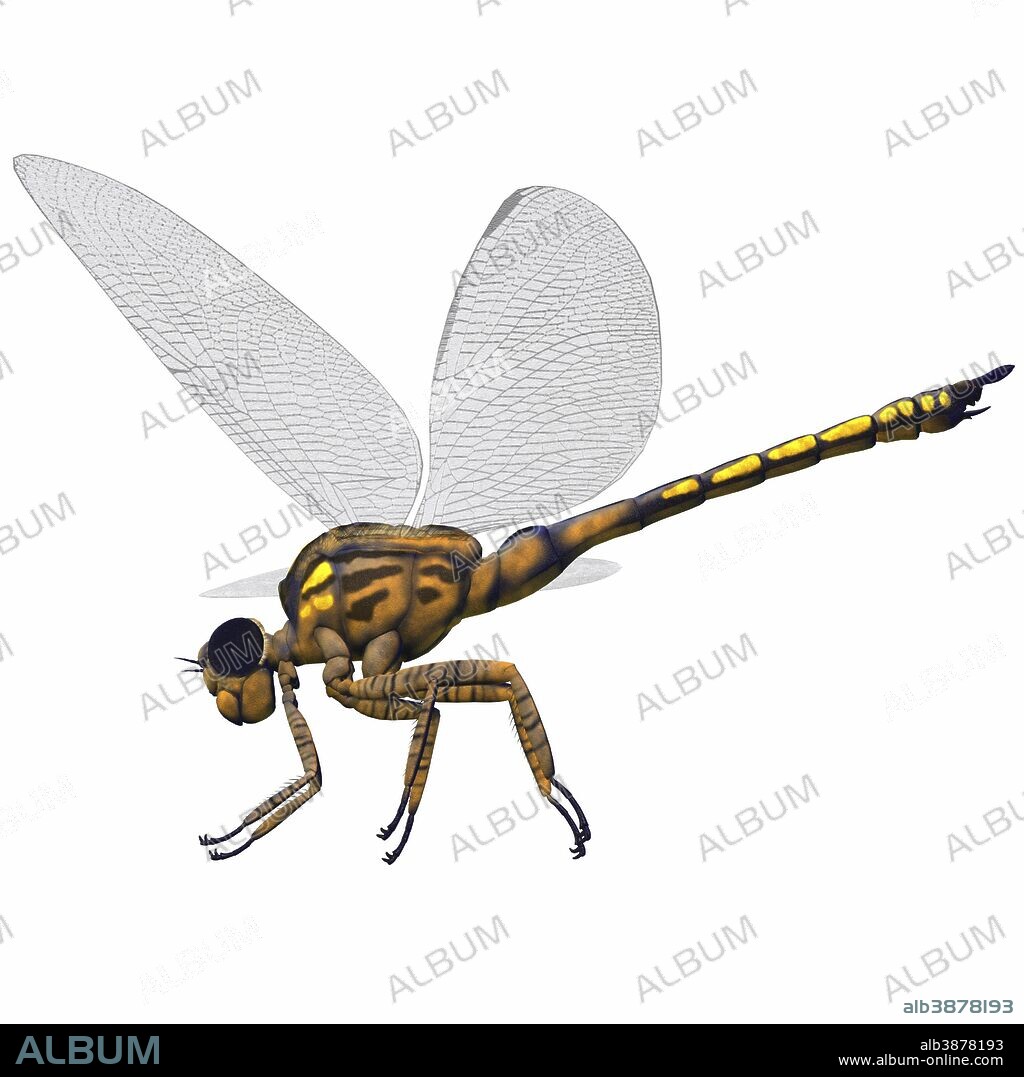This is a detailed visual representation of a dragonfly, set against a white background imbued with the word "album" repeatedly, mimicking a copyright watermark. The dragonfly, viewed from the side, showcases a segmented abdomen adorned in shades of brown, orange, and yellow, with dark blotches accentuating its form. The dragonfly’s long, elongated tail, continuing the orange with black accents and a yellow trim, juts out prominently. It has a typical dragonfly head with large black eyes and two small antennas. Its wings, four in total and appearing fairly broad and transparent, suggest readiness for flight. Below the insect, a black banner spans the bottom of the image. On the left within the banner, "album" is inscribed in teal, while the bottom right corner displays the code "ALB3878193" and the website "www.album-online.com."